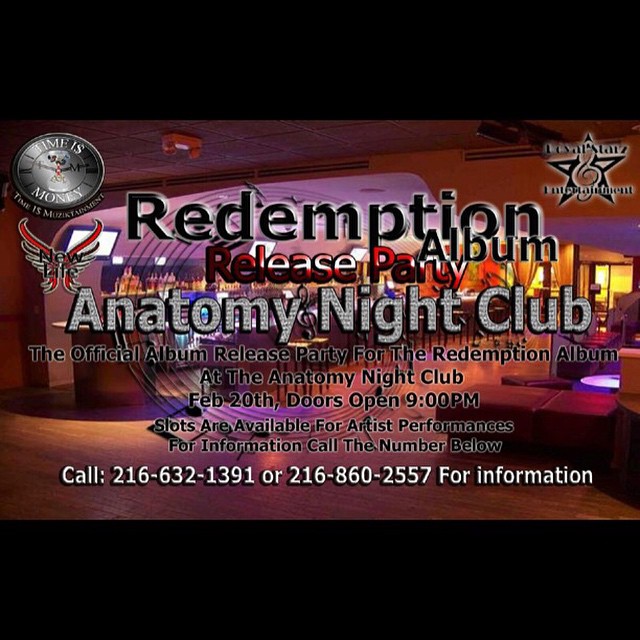The advertisement for the Redemption Album release party at Anatomy Nightclub is set against a backdrop of the nightclub’s interior during the day. The club is brightly lit with orange lights on the right side and purplish-white lights illuminating the bar on the left side. The venue features wooden floors, plenty of ottomans and seats, and numerous chairs against the bar, all contributing to its clean and stylish appearance. In the top left corner, a round icon with a clock and the phrase "time is money" adds a touch of flair, while the right side is adorned with a star-shaped icon containing a music note. Prominently displayed in large black text are the words "Redemption Album," followed by "Release Party" in red text, and "Anatomy Nightclub" in sparkling gray text resembling diamonds. The advertisement further details that the official album release party will take place at Anatomy Nightclub on February 20th, with doors opening at 9 PM. Slots are available for artist performances and further information can be obtained by calling the provided phone numbers: 216-632-1391 or 216-860-2557.